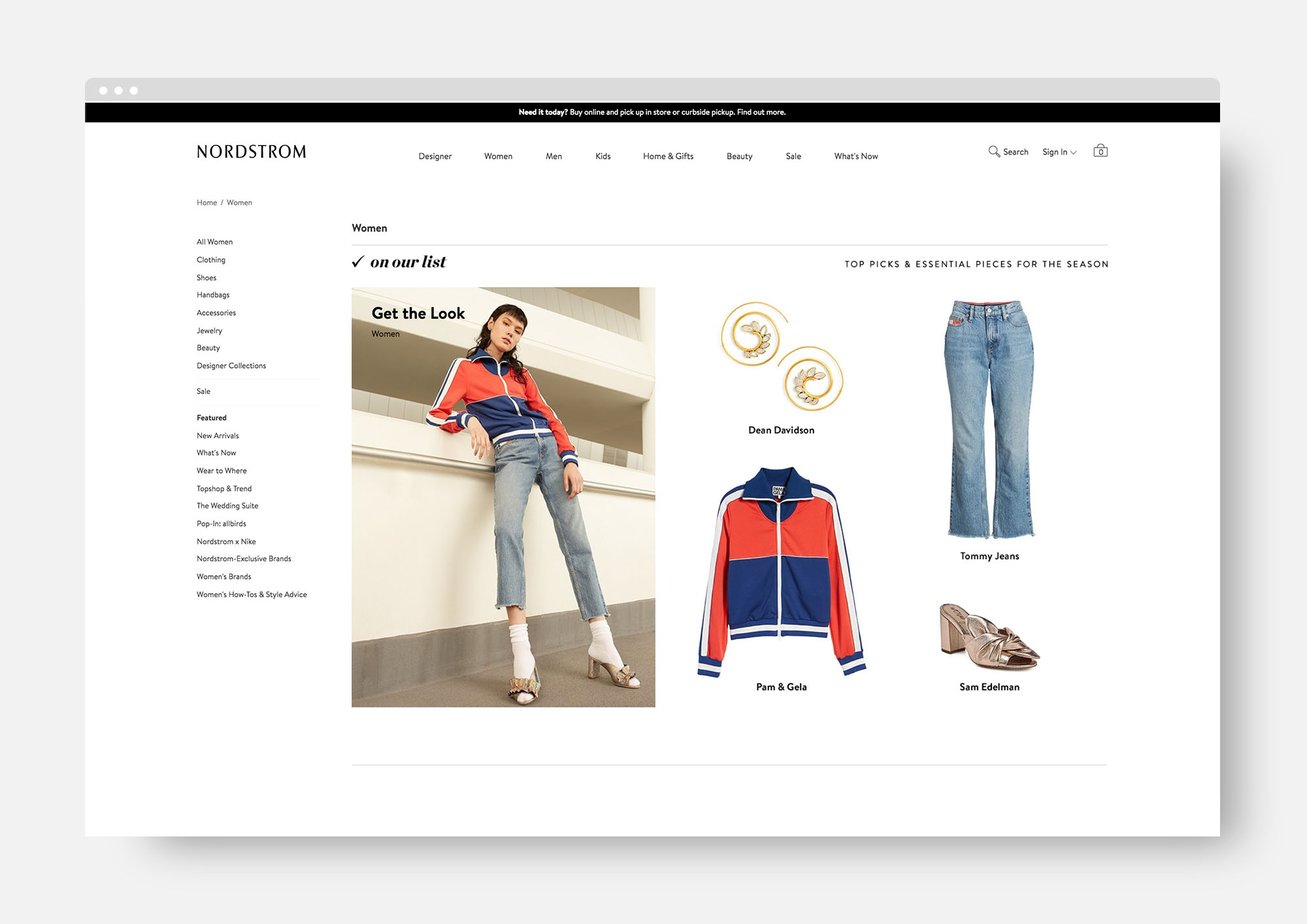In the screenshot of the Nordstrom website, we see a prominent black header with white text that reads, "Need it today? Buy online and pick up in-store or curbside pickup. Find out more." Below this header, the background turns white. In the upper left corner, "Nordstrom" is displayed in large, bold black text.

On the left side of the page, there is a navigation menu that includes the following categories: Home, Women, All Women, Clothing, Shoes, Handbags, Accessories, Jewelry, Beauty, Designer Collections, and Sale. Below these categories, under a bold black heading labeled "Featured," there are vertically listed subcategories: New Arrivals, What's Now?, Where to Wear, Topshop & Trend, The Wedding Suite, Pop-In: Allbirds, Nordstrom + Nike, Nordstrom Exclusive Brands, Women's Brands, Women's How-Tos & Style.

The main portion of the image showcases a color photo of a young woman leaning against a wall. She is dressed in denim jeans, white bobby socks paired with heels, and a sports jacket that features a combination of orange, blue, and white colors. Accompanying the image is the phrase, "Get the Look," positioned to the left of her head, tying into the navigational list.